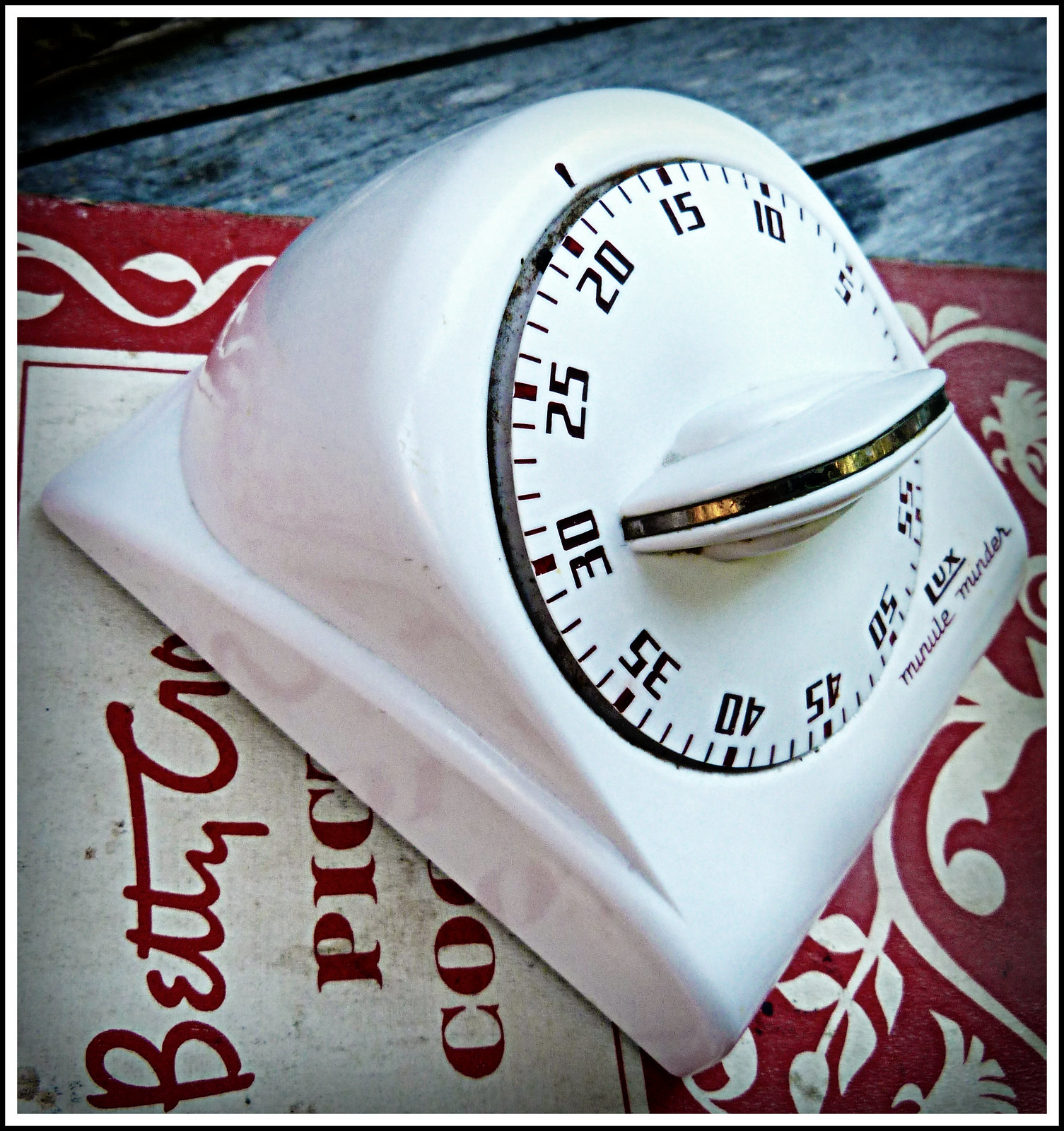This detailed color photograph features a close-up view of a weathered, gray wooden picnic table, possibly taken outdoors. The focus of the image is a vintage, red and white Betty Crocker picture cookbook, with notable cursive writing partially obscured by a Lux Minute Minder kitchen timer resting atop it. The cookbook showcases a red floral pattern against white cutouts, lending it a distinctly aged appearance with a worn, dirt patina. The timer, prominently displayed, is a white plastic device marked with numbers from 5 to 60, each separated by minute lines. It features a raised white handle with a metal and black trim running down the center, and "Lux Minute Minder" clearly labelled at the bottom.